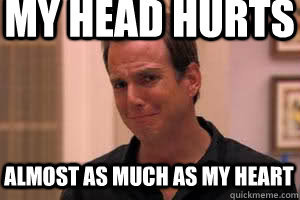The image showcases a very muscular, middle-aged man, likely between 40 and 45 years old, positioned on a bed in a suggestive manner. He sports a faded tattoo on his right shoulder featuring a star and laurel leaves, and has a very hairy chest along with a short beard and balding head. The man is clad in a black jockstrap, straddling a cylindrical pillow that matches the bed's decor, which includes a black, gray, white, and red camouflage-patterned bedspread. He is gazing intensely at the camera while on his knees with legs spread towards the bed.

The bedroom setting is quite luxurious, featuring a rich, dark chestnut stained poster bed set against a shimmery textured charcoal gray wallpaper. The bed is adorned with black satin pillowcases, with distinctive white stripes on either end, and the camouflage-patterned pillow positioned in the middle. Electrical outlets are visible on either side of the bed, though nothing is plugged into them. At the bottom of the photo, the text "H-A-I" is prominently displayed. The overall atmosphere suggests that the image could potentially be an advertisement or meme, possibly related to adult industry content. The dimensions of the image are approximately nine inches across by six inches tall.